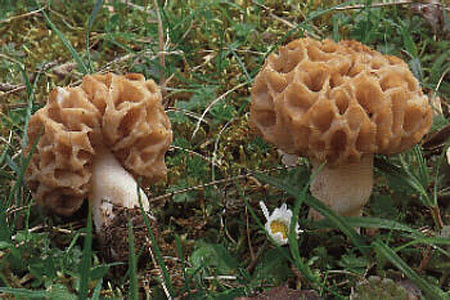This detailed image captures a close-up outdoor scene from ground level, prominently featuring two morel-like mushrooms amidst a dark grassy background. The left mushroom lies on its side, revealing its dirt-covered white stalk, and neighboring a patch of exposed soil. The standing mushroom to the right showcases a creamy base transitioning into a light orange-gray, porous cap resembling a sponge or coral with large grooves. Between these fungal figures stands a daisy, its yellow center surrounded by yet-to-open white petals, juxtaposed against blades of green and yellow grass and a small area of dirt. The unique, flat-topped mushrooms appear almost like a mosaic of cells, creating an intricate texture across their caps.